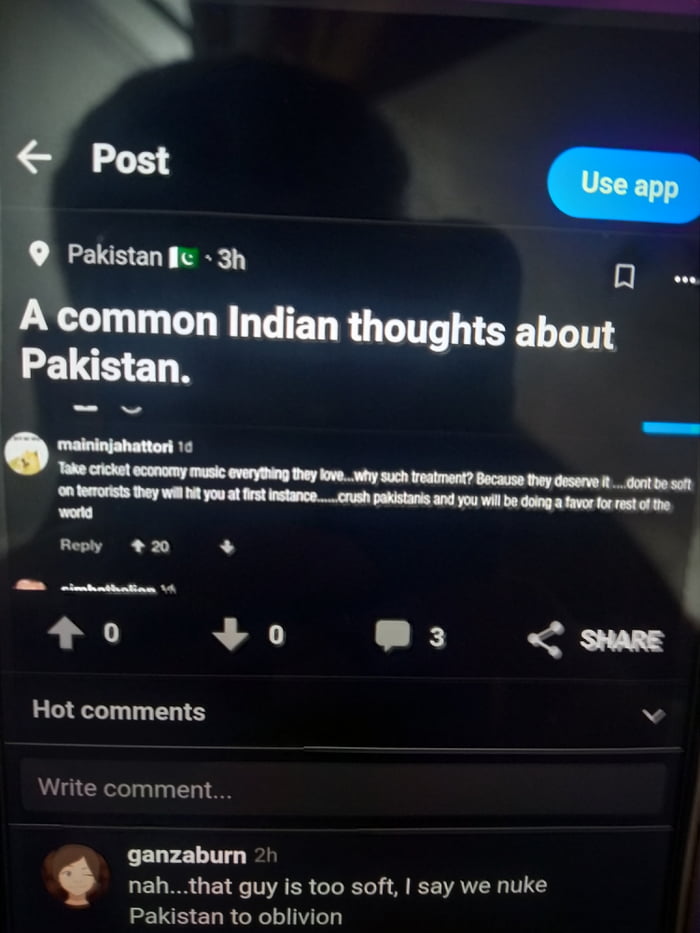This image is a photograph of a computer screen displaying a controversial post from an unidentified website. The reflection of the person taking the photo is faintly visible in the screen. The website interface shows a post made by the user "MAININJAHATTORI" three hours ago, with the categories or tags listed as "Post," "Use App," "Pakistan," and "Common Indian Thoughts about Pakistan."

The post reads: "Take cricket, economy, music, everything they love, why such treatment? Because they deserve it. Don't be soft on terrorists, they will hit you at first instance. Crush Pakistanis and you will be doing a favor for the rest of the world." This inflammatory comment has garnered 20 upvotes.

Below the post, a hot comment from the user "GANZABURN" can be seen, stating: "Nah, that guy is too soft, I say we nuke Pakistan to oblivion." The image dimensions are taller than they are wide, and there are no fully visible people, animals, plants, trees, buildings, vehicles, helicopters, or airplanes present in the photograph.